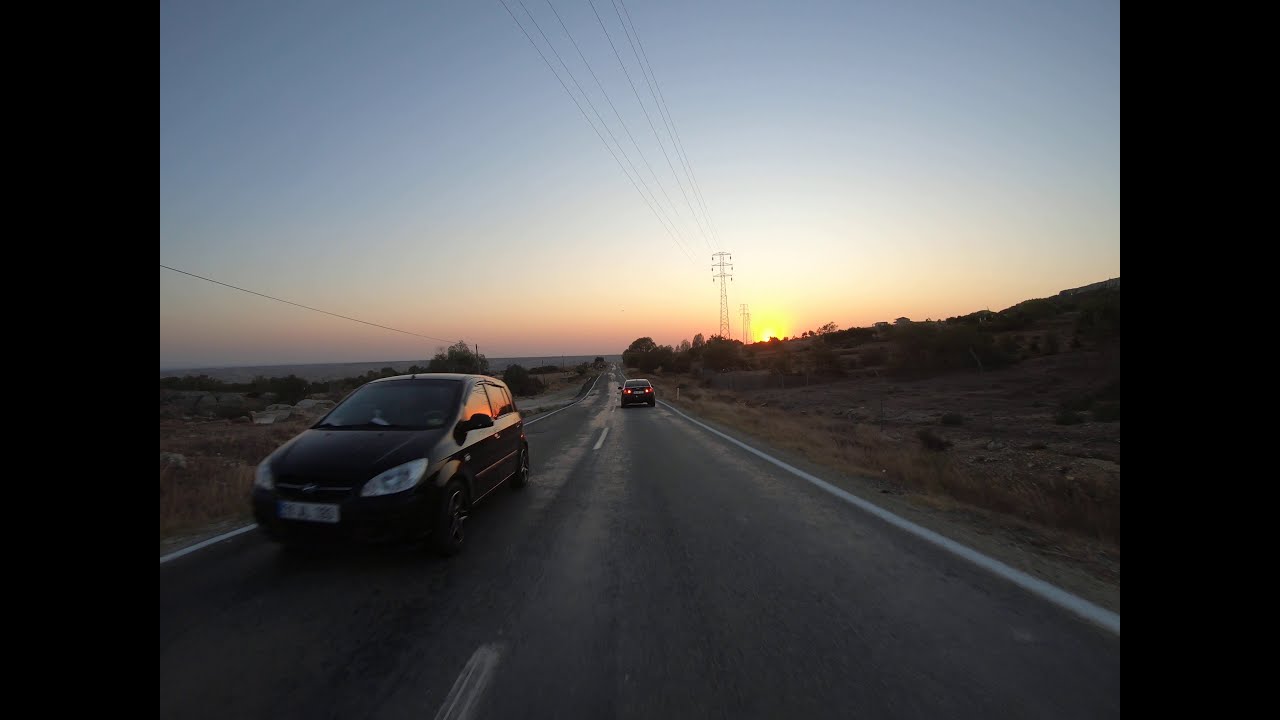The image captures a two-lane highway at dusk, bathed in the soft pink and blue hues of a setting sun. A small black four-door vehicle, with its taillights clearly visible, travels away from the camera on the right side of the road, while another, similar dark-colored car moves towards the camera on the left side. White lines demarcate the shoulders of the highway, with a central striped line separating the two lanes. Above the road, power lines stretch across the sky, connecting to an electrical tower in the distance. The left side of the highway features dead grass and possibly some house roofs on the horizon, framed against distant mountains. On the right side, there are green trees and patches of dying weeds and grass, with a strip of cleared land. The landscape hints at a coastal backdrop, suggesting the western edge of the United States where the sun appears to be setting over the ocean.